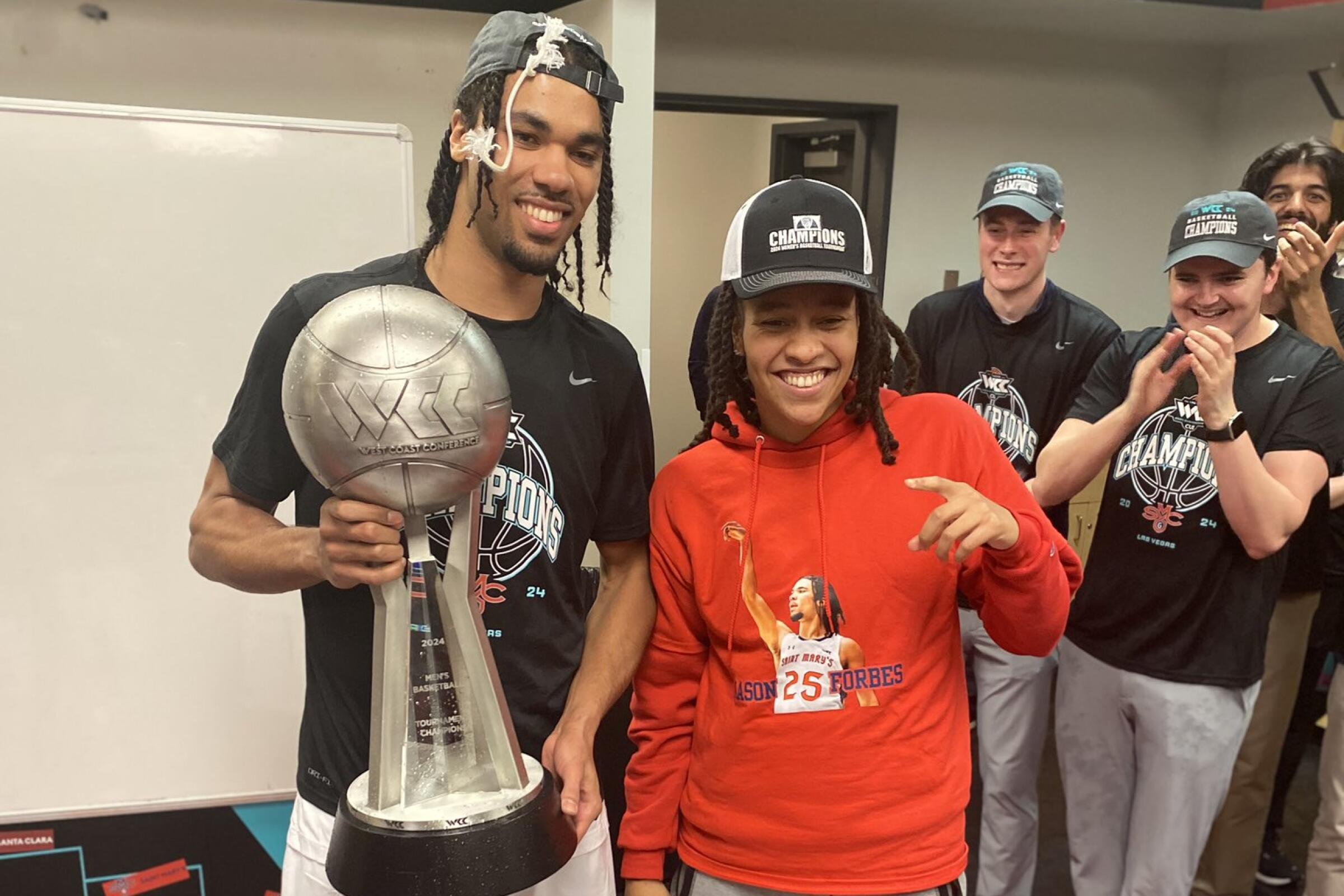In this celebratory locker room photograph at St. Mary's College, a tall basketball player on the left proudly holds a trophy topped with a silver basketball, both bearing the "WCC Champions" inscription. He is donning a black t-shirt also emblazoned with "WCC Champions" and the St. Mary's College logo. Beside him is a person in a distinctive red sweatshirt featuring the name "Mason Forbes" and a photograph of the wearer. In the background on the right, several other players wear matching black championship t-shirts and hats, clapping and smiling, adding to the joyful atmosphere. The locker room's features, including a clean whiteboard and an open door, frame this victorious scene.